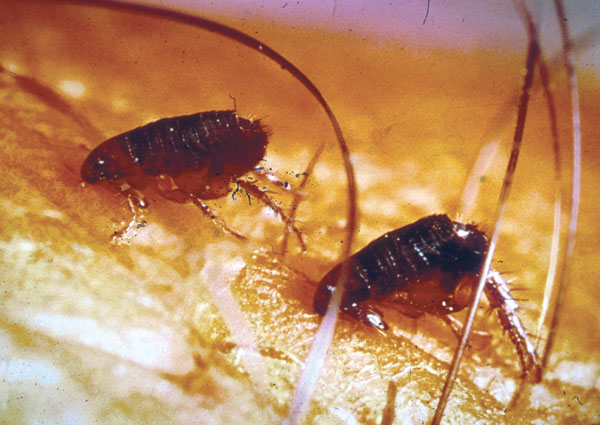The close-up rectangular photograph, approximately four to five inches wide and three inches high, reveals a microscopic view of two dark brown fleas on what appears to be human skin. The image, illuminated from the lower left, slants from the upper left corner to the lower right, casting an orange tinge across the surface. The skin is very light, adorned with long brown hairs that transition from white at the base to brown at the tips. The fleas are aligned one above the other, facing left, with their darker backs contrasting their slightly lighter, silvery legs. Their mouths are bent down and appear to be biting into the skin, with their heads in a lighter brown shade compared to their darker bodies. The fleas' long legs showcase visible bends and are covered in fine hairs, adding to the overall eerie and detailed ambiance of the image.